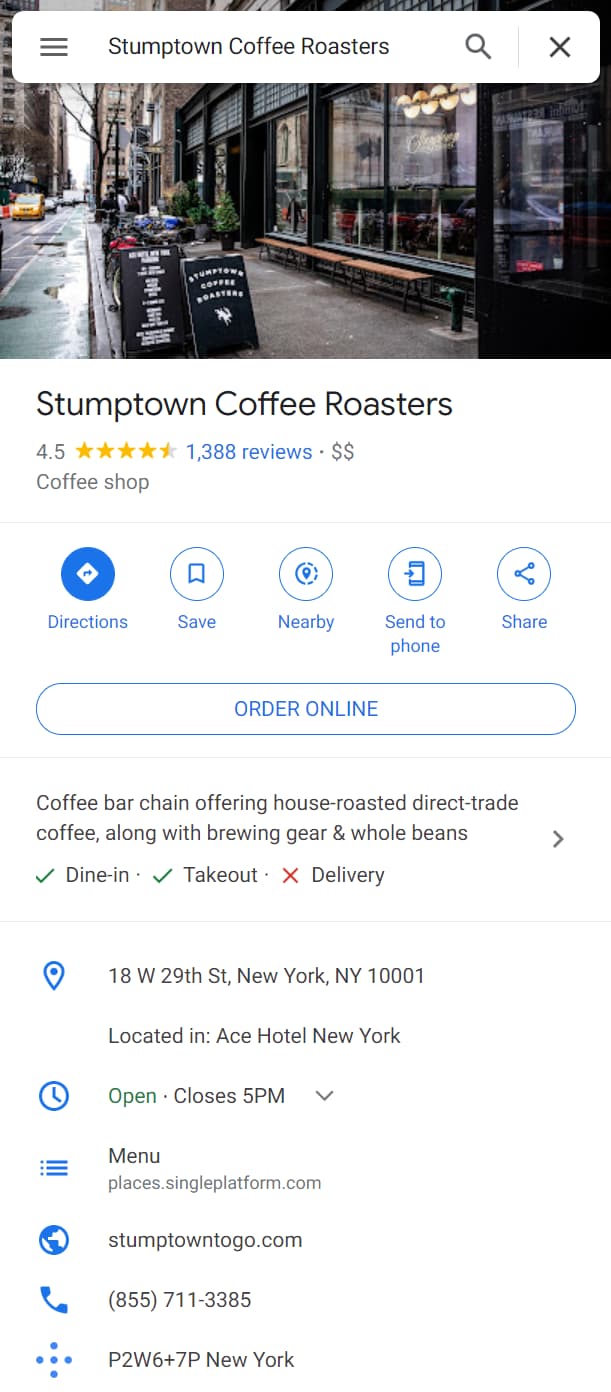The screen capture from a mobile device displays a search bar at the top with the phrase "Stumptown Coffee Roasters" and a search icon to the right. Directly beneath the search bar is an image showcasing the exterior of a café or restaurant, featuring large windows and monochromatic signage on the sideboard beside the street. A yellow taxi cab is visible in the background on the left side of the image. Below this picture, "Stumptown Coffee Roasters" is prominently written, followed by a rating of 4.5 out of 5 stars, with the fifth star half-filled. Additionally, it indicates there are 1,388 reviews in blue text. At the bottom portion of the screen, there are icons for directions, saving the location, finding nearby places, sending the location to a phone, and sharing. There is also a blue button labeled "Order Online".